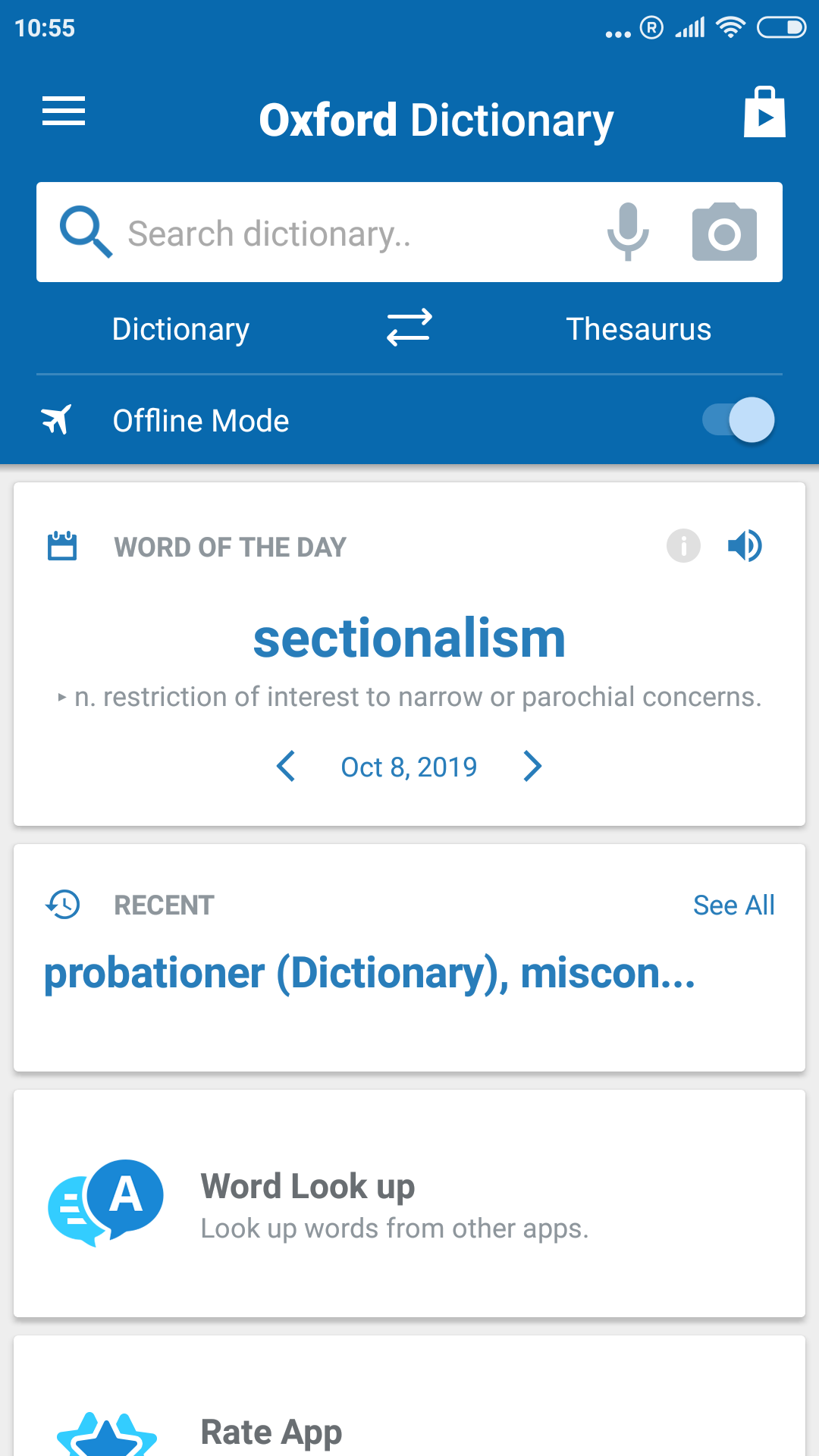The screenshot features an interface from the Oxford Dictionary app. In the top left corner, the time is displayed as "10:55" in white. Dominating the center is the "Oxford Dictionary" title, accompanied by a search bar. This search bar includes a blue search icon, along with gray icons for a microphone and a camera. Below this, the sections are divided with "Dictionary" and navigational arrows for viewing previous and next sections, flanked by "Thesaurus" on the right.

Further down, an airplane icon indicates "Offline Mode," with a toggle switch positioned to the right, indicating that it is activated. The "Word of the Day" section follows, presenting "sectionalism," defined as "restriction of interest to narrow or parochial concerns." This section includes navigational arrows dated "October 8, 2019," allowing the user to browse between different words of the day.

The screenshot also lists recent searches: "probationary (dictionary)" and "MISCON." At the bottom, there's a "Word Lookup" section with an option to rate the app.